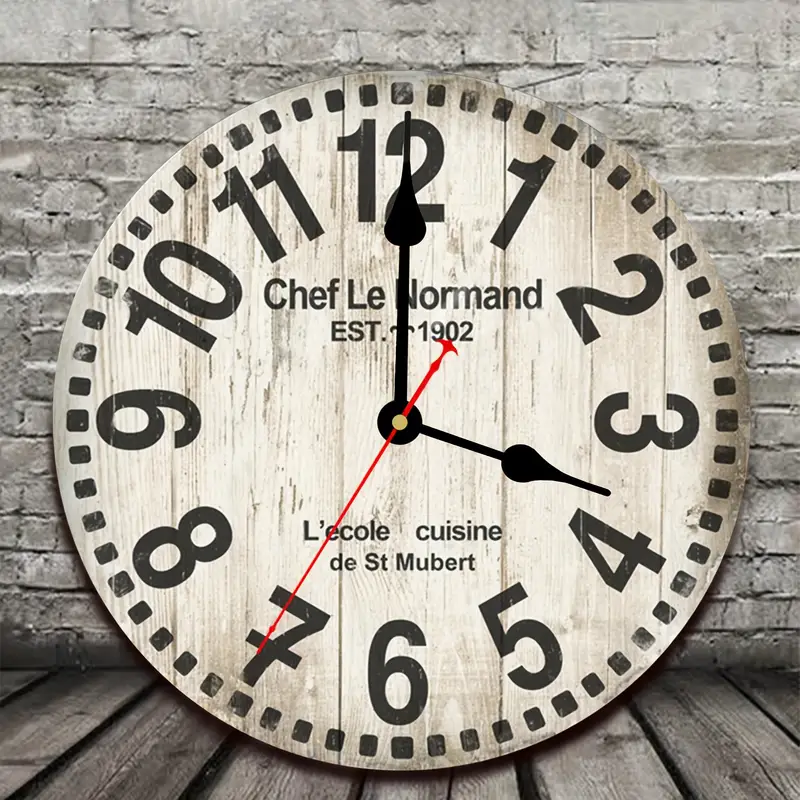The image showcases a large, round, decorative clock with a rustic gray wooden finish, placed against an old brick wall backdrop. The clock is set on wooden panels with visible gaps, suggesting it's either on a floor or table. Its black and gray design features large, prominently displayed numbers from 1 to 12 and small dots marking each second around the circumference. The clock reads four o'clock, with the minute hand being red, and sits directly on the 7. An inscription at the top reads "Scheffler Normand established 1902," and another at the bottom reads "Le Col Cuisine de Saint-Mubert." Despite its realistic appearance, there are hints that this could be a photoshopped image or a graphic design work given its meticulous details.